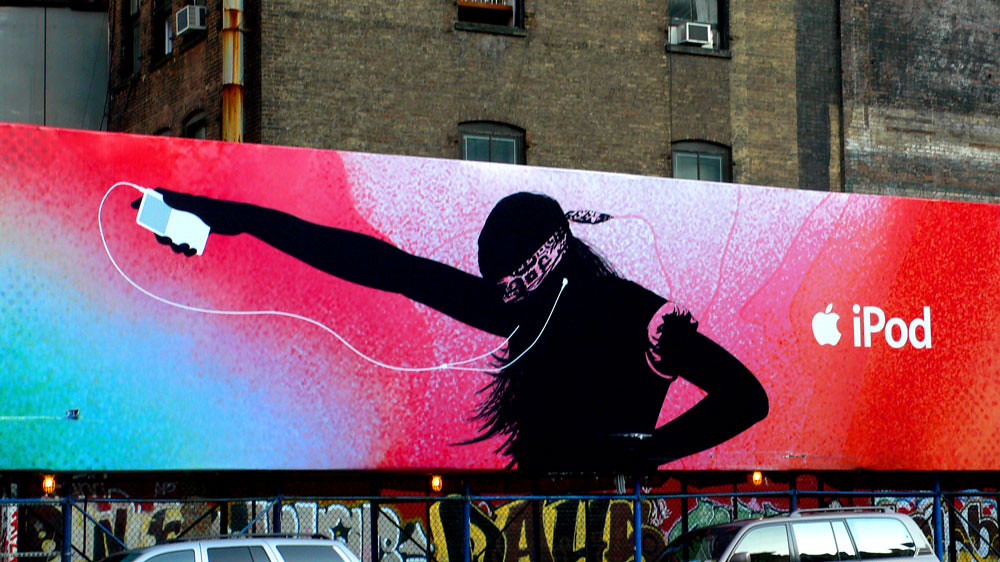A vibrant and large billboard stands prominently in a densely populated urban neighborhood, possibly in the Bronx. Behind it, an old apartment building looms, identifiable by its lack of central air conditioning as evidenced by window units on the third floor. The billboard, a striking contrast to its surroundings, exudes a bright, happy, and energetic vibe. It stretches across the wall, which is adorned with extensive yet illegible graffiti, and features a secure blue gate at the base. Parked nearby are two vehicles—a silver minivan and a gray hatchback.

The billboard itself is an eye-catching advertisement for iPods, showcasing a gradient color scheme transitioning from green to blue, to red-pink, and then a light pink, culminating in red. At the center of the billboard is the silhouette of a woman, radiating energy and dynamism. She stands with her right arm fully extended, clutching an iPod, with its iconic white earbuds trailing down. Her left arm rests confidently on her hip, and both of her sleeves are rolled up, revealing a pink color. The woman's bandana, in pink and black, ties back her hair, which streams down toward her waist, animated as if she's dancing. The overall aesthetic suggests a fusion of happiness, modernity, and perhaps a hint of hip-hop culture, effectively capturing the lively essence of the brand.